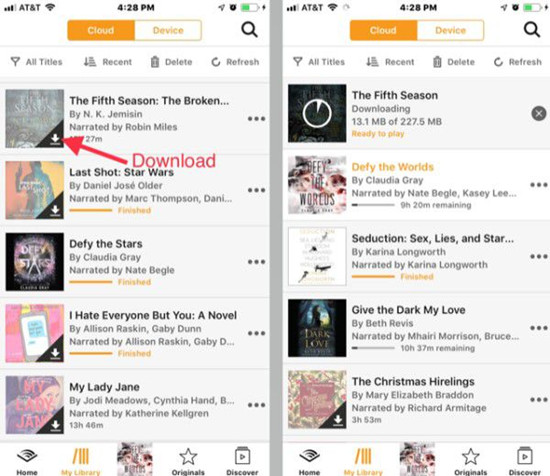The image showcases two screenshots from an iPhone running on AT&T service, with the time displayed as 4:28 PM and the battery level at half green. The first screen displays a title bar labeled "Cloud" and "Device," with the cloud option highlighted in orange. Below, there's a navigation bar with options for "Old Titles," "Recent," "Delete," and "Refresh." On the left side of this screen, there are images resembling book covers. The first cover features a prominent red arrow pointing to it, identifying it as "The Fifth Season" with the subtitle "The Broken," and the text "Download" in red lettering.

The second screen similarly features "The Fifth Season" at the top, indicating that the item is currently "Downloading" and "Ready to Play" in orange text. Beneath this top item, additional selections can be made. At the bottom of each screen, there are icons representing different menu options: a phone, "My Library" highlighted in yellow, a graphical image, "Originals" with a star icon, and "Discover" featuring a box with an arrow.